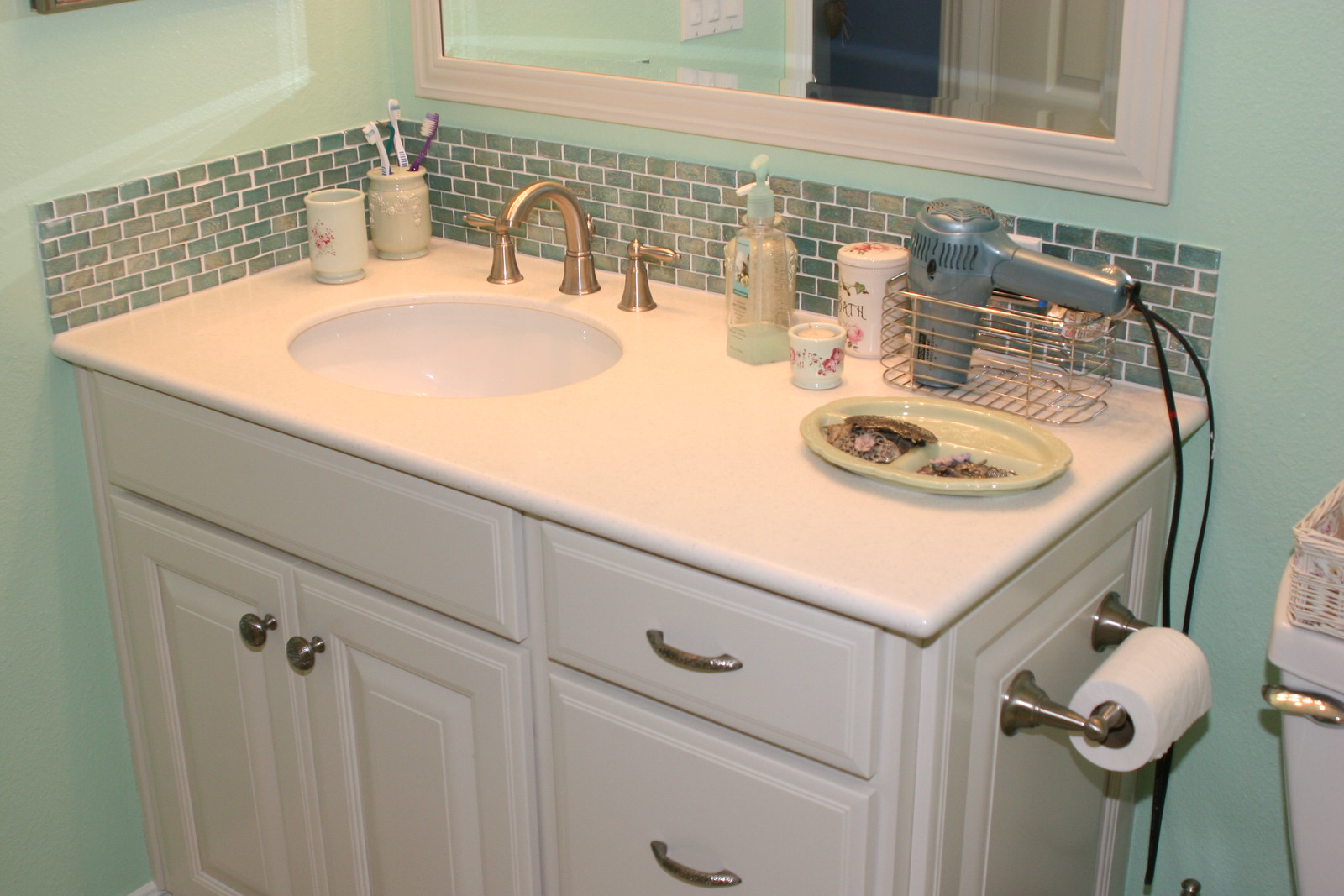The color photograph captures a well-lit bathroom countertop adorned with a stylish tile backsplash, featuring a harmonious blend of green, gray, and white tiles, separated by pristine white caulking. The backdrop of this striking backsplash is set against calming light green walls. Mounted on the wall, above the countertop, is a sleek, flat mirror, reflecting parts of the room that extend beyond the photo's frame.

On the left side of the white laminated bathroom counter, near the sink, a white ceramic cup holds three toothbrushes. Beside it sits an empty cup, likely intended for rinsing. The sink itself boasts sterling silver fixtures that add an elegant touch. Positioned to the right of the sink is a pump bottle, possibly containing hand soap, though the label is obscured and not readable. 

Adjacent to the pump bottle is a stainless steel basket containing a hairdryer. A white circular plate with three compartments is also present, although the contents of two compartments remain indistinguishable, with one compartment notably empty. Below the sink, the cabinetry is highlighted by sterling silver knobs, hinting at a cohesive design aesthetic.

To the right of the vanity, a mounted toilet roll holder provides easy access to toilet paper. The edge of a white toilet with a stainless steel handle is visible at the far right of the image, partially cropped out, leaving the full picture of the back of the bathroom to the imagination.